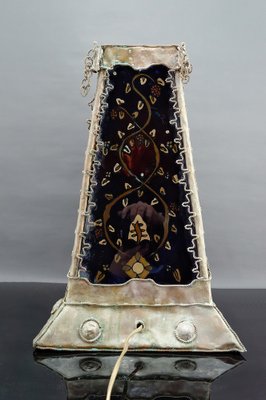The photograph features a vintage, metallic, metronome-shaped object against a light gray wall background, with a darker gray to black tabletop. The object, possibly a lamp, has a trapezoidal form that is wider at the bottom and narrower at the top, giving it a distinctive tapered structure. The base is a broad, flat trapezoid, above which another skinnier trapezoid sits. This top portion showcases intricate designs, with an orange-brown pattern resembling DNA-like squiggly lines in the center, bordered by a white patterned ridge on either side. Surrounding these central designs are numerous U or V-shaped symbols in a light white-tan hue. The metal appears somewhat tarnished and rough, adding an aged, vintage aesthetic. A cord extends from a hole at the bottom center, indicating it might require electricity. Additionally, there are two circular buttons or covered holes at the base, contributing to its intricate design.